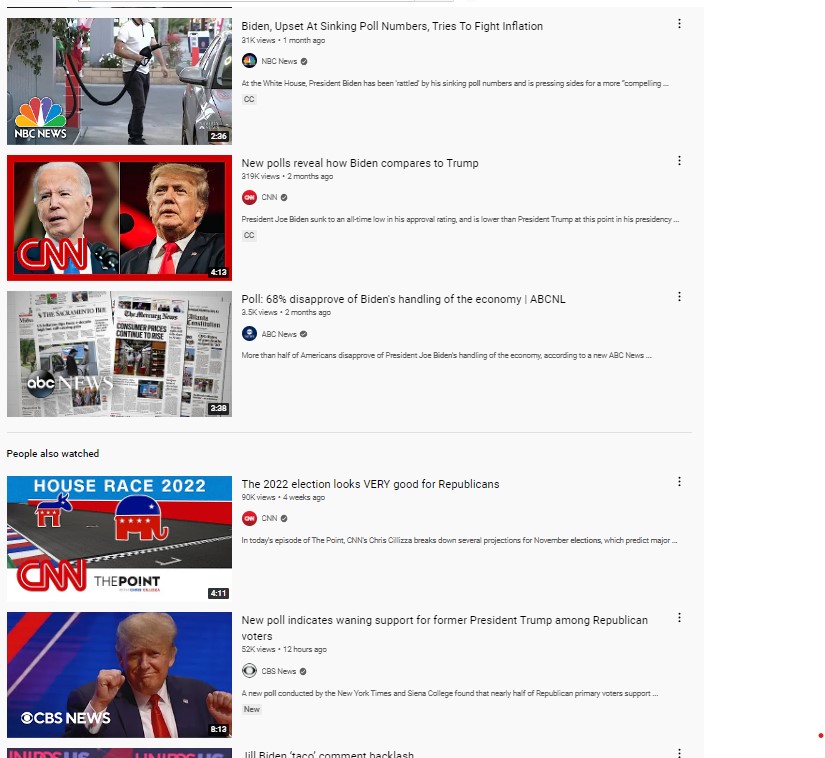Screenshot capturing prominent news articles from various networks. The first article, from NBC, features an image of a man pumping gas next to the iconic NBC peacock logo. The second article, by CNN, displays photos of President Biden and former President Trump under the headline "68% Disagree with Biden’s Handling of the Economy." The screen also showcases a poll graphic from ABC regarding the 2022 House races, highlighting ongoing coverage and analysis. The assortment of articles represents the extensive media focus on political and economic issues leading up to the 2022 elections.